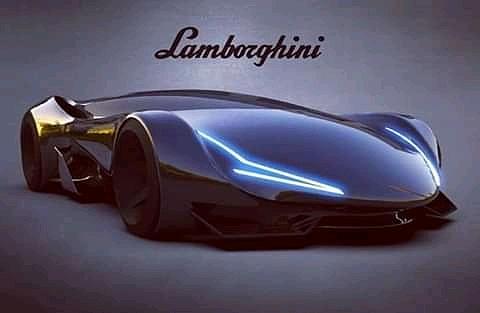The advertisement prominently features a sleek, futuristic Lamborghini that appears to be either a concept model or a very limited production run. The car, likely computer-generated or a prototype, is depicted in stark, striking detail. Above the vehicle is the iconic Lamborghini font and logo, simply reading "Lamborghini." The car itself is black with vivid neon blue headlights and black wheels. Its ultra-low, cyberpunk-esque design is characterized by the hood flowing seamlessly into the rear, with no apparent cab. The fenders are higher than the car body, giving it a laid-back, aerodynamic profile. Unique design features include a protruding iron-like front bumper and rear air intakes positioned just above the fenders. The car's long, triangular front lights add to its cutting-edge appearance. Set against a black and light gray background, the image is clear and brightly lit, focusing entirely on the car with no other vehicles, people, or text present.